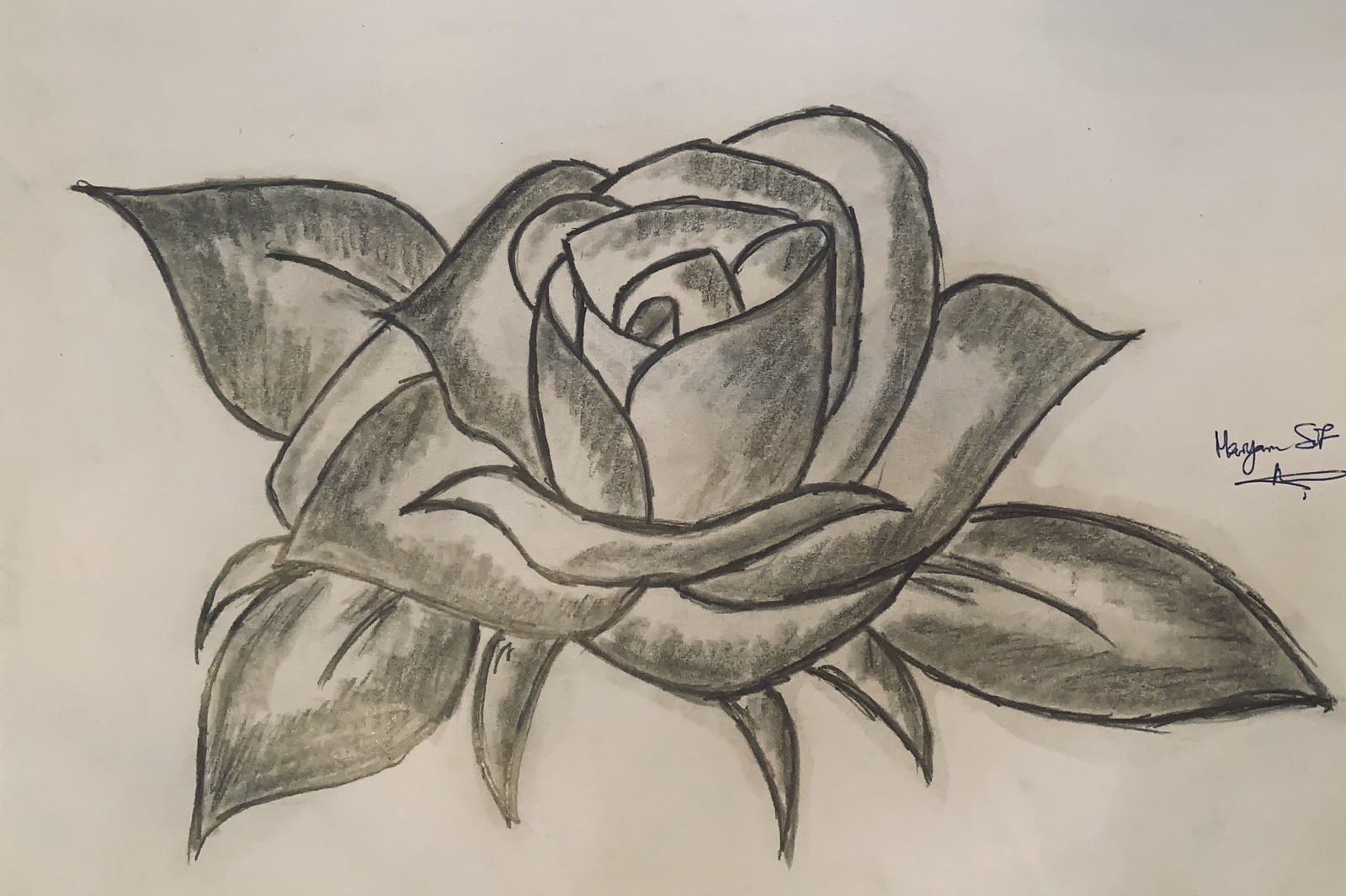The image depicts a meticulously hand-drawn pencil sketch of a rose on a rectangular white piece of paper. The lines of the rose petals and the three surrounding leaves—two on the left and one on the right—are marked with a bold, intense black, possibly indicating the artist may have initially outlined the sketch with a black marker before finishing it with pencil. The shading is skillfully applied, with darker smudge marks accentuating the edges and providing depth, while the interiors of the petals and leaves are lighter, enhancing the texture and realism of the drawing. At the base of the flower, three prongs of the sepal are visible, adding to the anatomical detail. The paper appears to have some smudge marks likely from the artist's hand. In the center-right area of the drawing, there is a cursive signature that looks like it could start with an "H" or an "M" and reads something like 'Marianne SF' with a squiggly line beneath it.